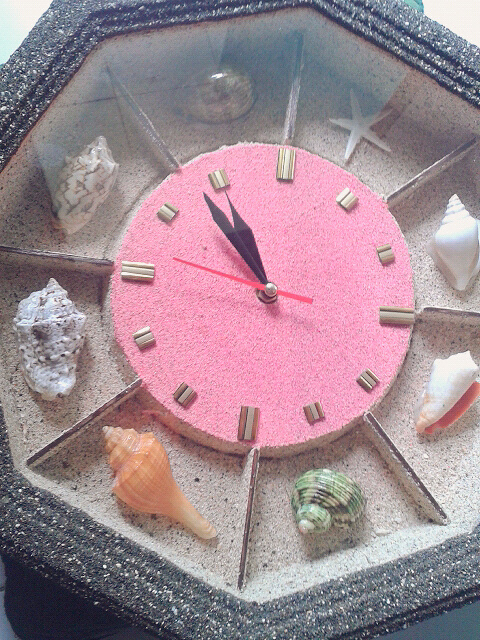This detailed image depicts a clock with a distinctive octagonal case, featuring a rough black border with specks of white scattered throughout. The clock face showcases a sandy texture adorned with an array of seashells, each marking the hours from one through twelve. At the very center of the clock, a prominent, sand-textured pink circle stands out, appearing three-dimensional with its vibrant color.

The hour markers are crafted from either silver or gold chunks of material, possibly wood or metal, giving the clock a rustic yet elegant look. The timekeeping hands are of contrasting colors: the hour and minute hands are black, while the second hand is vivid red. The clock face is segmented with dividers corresponding to each seashell position.

Among the seashells, there is a variety of forms and colors. Starting from one, a shiny, rounded shell is visible, followed by a small white starfish at two. At three, a tiny, swirled white shell is placed, while at four, a conch shell with a pink interior is displayed. Moving to five, a green and white shell with black indentations stands out, and at six, a peach-colored swirled shell appears. Seven to twelve involve shells that vary from white with brown accents to shiny white with brown details. Underneath these shells, the sand creates a consistent and natural backdrop, while the dividers, resembling pieces of wood, emphasize the separation between each unique shell.